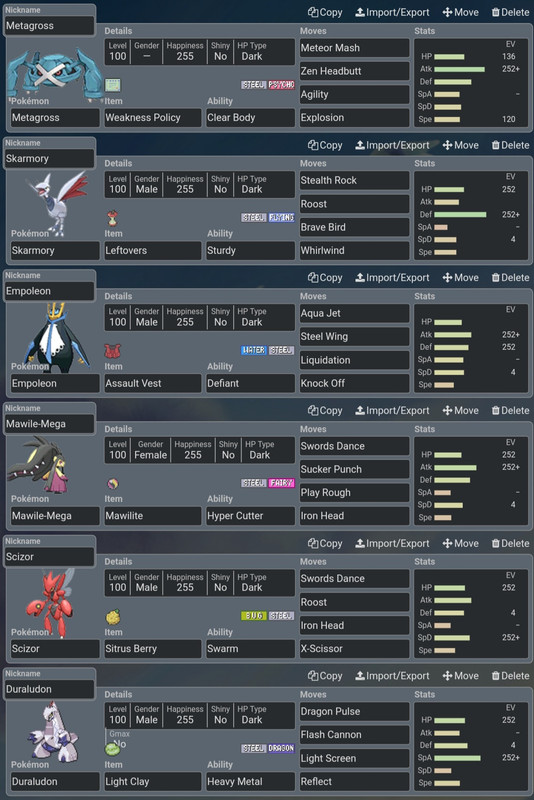This image is a detailed screenshot from a Pokémon character guide, focusing on a character named Metagross. The screenshot is set against a gray background, with each Pokémon character displayed on its own individual tab. There are a total of six tabs visible at the top of the screen. At the top right corner, functional buttons labeled "Copy," "Import," "Export," "Move," and "Delete" are present for managing the character data.

Metagross, featured prominently at the top, exhibits its moves and statistics, clearly indicating it as the strongest character among the six. Metagross's impressive stats are outlined, suggesting its supremacy. In contrast, the second character shown, which appears to be Skarmory, resembles a bird and seems to possess the weakest stats among the displayed Pokémon. This visual comparison highlights Metagross as the overall best performer in the guide while suggesting that Skarmory is the least powerful.